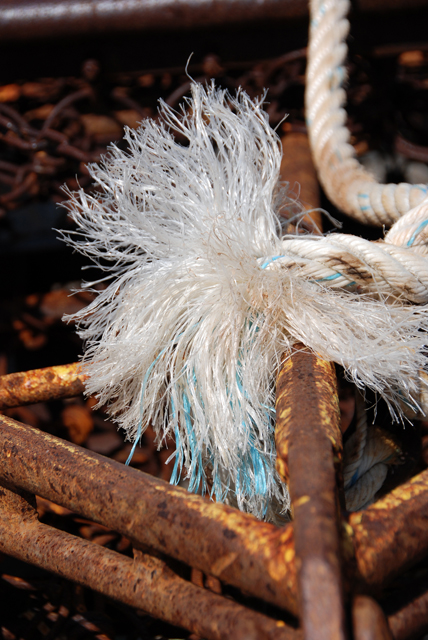In the center of the photograph is a heavily frayed white rope with light blue strands woven into it, the frayed end splaying out in an inch or two of tangled fibers. This rope extends back toward the upper right-hand corner of the image, where the rest of it is visible, displaying its white color interspersed with light blue strands. The rope is draped over and resting on what appears to be a rusted metal basket or container, characterized by its brown rust coloration. Additionally, a long, indistinct pole-like object lies atop this rusted structure. The background is filled with various rusted metal objects, lending a dark, decrepit, and industrial atmosphere to the scene reminiscent of an old, rusted basement.